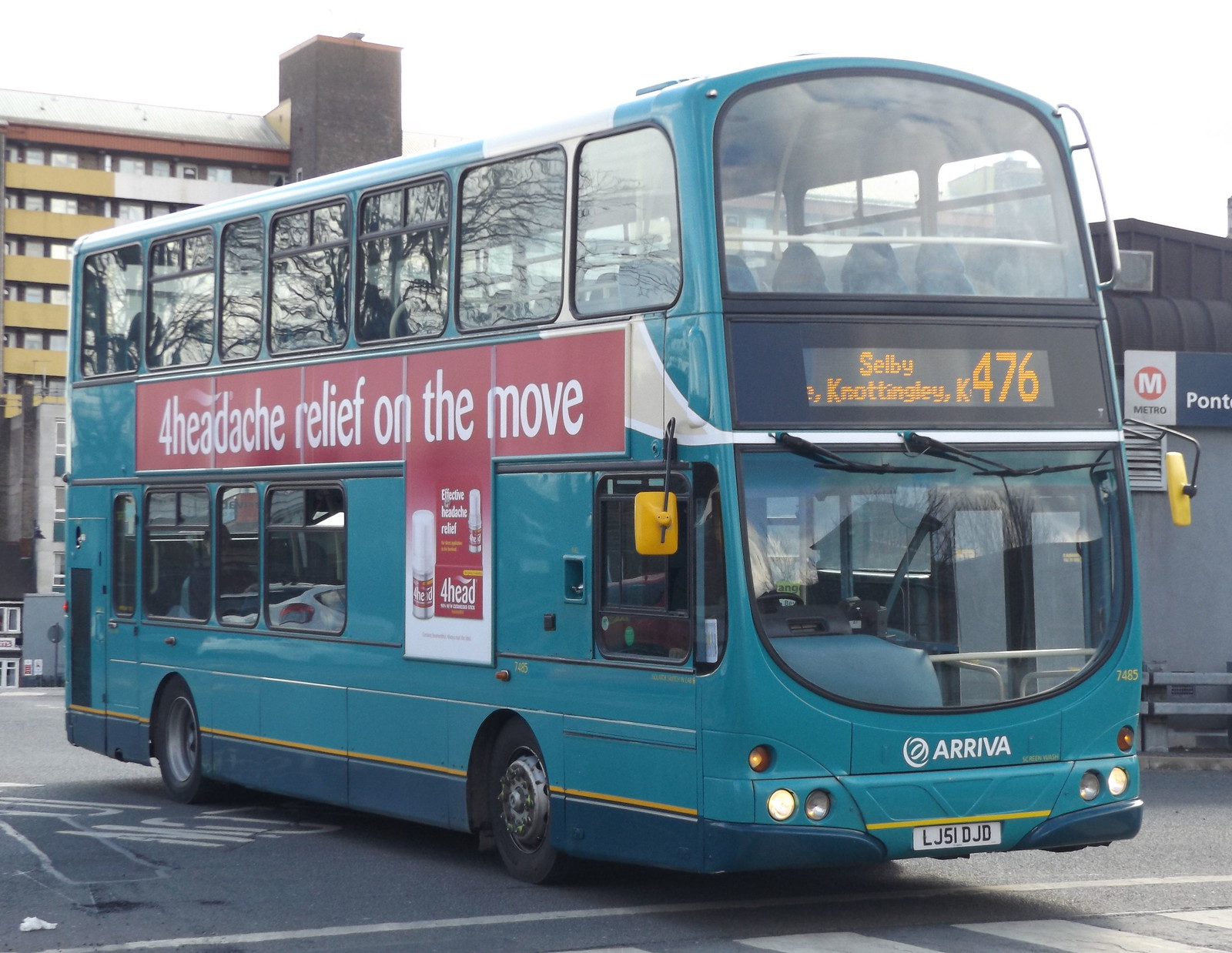This image captures a static, double-decker bus prominently featured in the foreground. The bus, which fills the entire frame, sports a two-tone blue color scheme: a light turquoise blue covers the upper portion, while a darker blue decorates the lower section around the tires. Yellow covers the side mirrors, adding a contrasting accent. Inscriptions adorn the vehicle: on the left side, a red banner with white font advertises a product called AHEAD, stating, "For Headache Relief On The Move," with an image of the medicine hanging below the text. The front electronic display reads "Selby, Nottington, K476," which appears to indicate the bus route, along with the license plate number LJ51 DJD. The iconic ARRIVA logo is displayed beneath the large windshield.

The bus is positioned slightly diagonally, with its front right side angled towards the camera and the back left barely visible. The image captures the top deck’s large front window and mirrors on the right-hand side of the bus. The scene is set outdoors under a white sky, suggesting an overcast day. No people are present around or inside the bus. The ground is grey, showing driving marks, and neither building in the background is distinctly identifiable. The left backdrop features what looks like a six-story apartment building, while on the right, part of a smaller building with a letter "M" on a gray wall and dark roof is visible. A small fence can also be seen on the far right. Despite the buildings, the bus remains the undeniable focal point of the image.